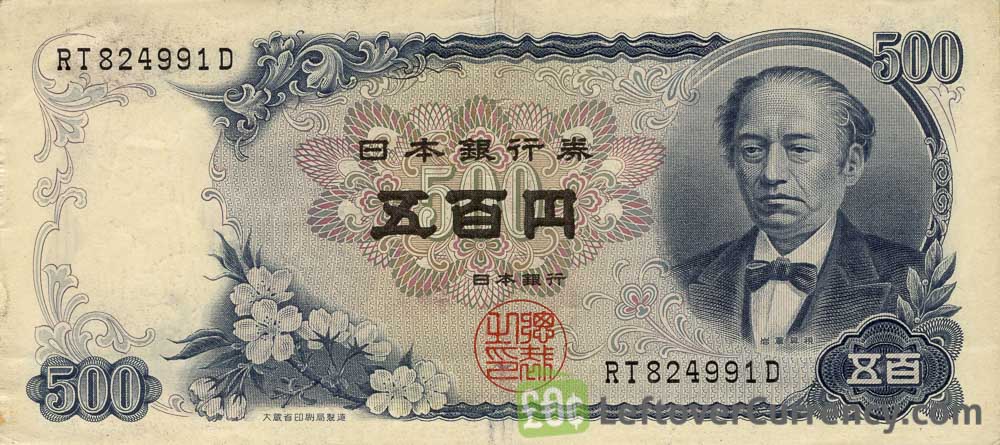The image depicts a well-preserved banknote from an unspecified Asian country, likely an old 500-yen bill, characterized by its light pink paper and blue and sepia tones. Central to the bill is text in an Asian language, possibly Mandarin or Japanese, prominently overlaid with the number "500." The number "500" is also repeated in the bottom left and top right corners. On the right side of the bill is the portrait of an elderly gentleman with short, swept-back dark hair, a tall forehead, and a drooping chin. He is dressed in a dark suit, white dress shirt, and black bow tie. A floral pattern adorns the border of the bill, adding to its detailed design. The banknote also features black lettering "RT 824 991 D" in the upper right corner, a green stamp with "zero pound cent," and a red circle with additional Asian characters in the lower center.